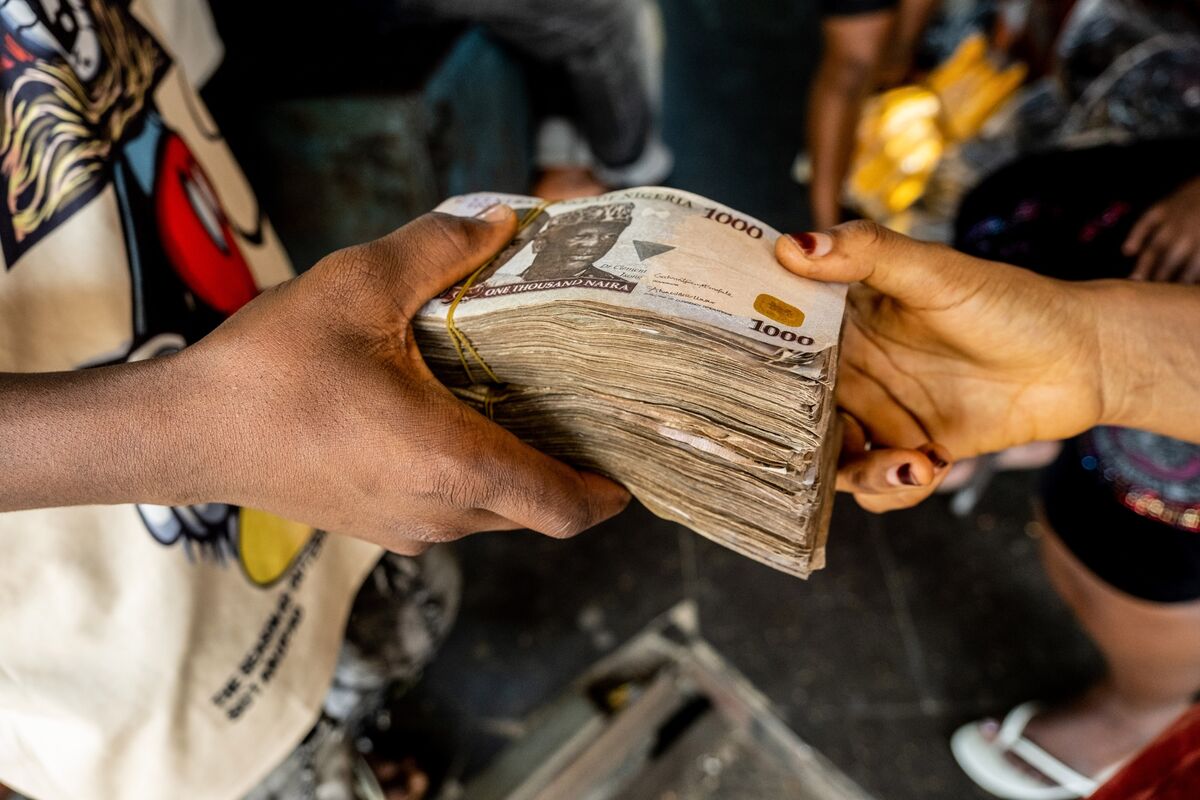In this close-up photograph, we see a detailed exchange of a large stack of 1,000 Naira notes between two individuals. The hands are prominently featured: one hand, which appears to belong to a man due to its larger size and lack of nail polish, is holding and possibly handing over the money. He wears a white t-shirt with a prominent Mickey Mouse character on it. The other hand, likely belonging to a woman, is characterized by smaller fingers with chipped red nail polish, suggesting it needs a manicure. The currency depicted shows a black man's image and features a grayish-blue and beige design with a gold stamp. In the background, partially visible, is a person wearing white thong slippers and black shorts, adding context to the scene's environment.